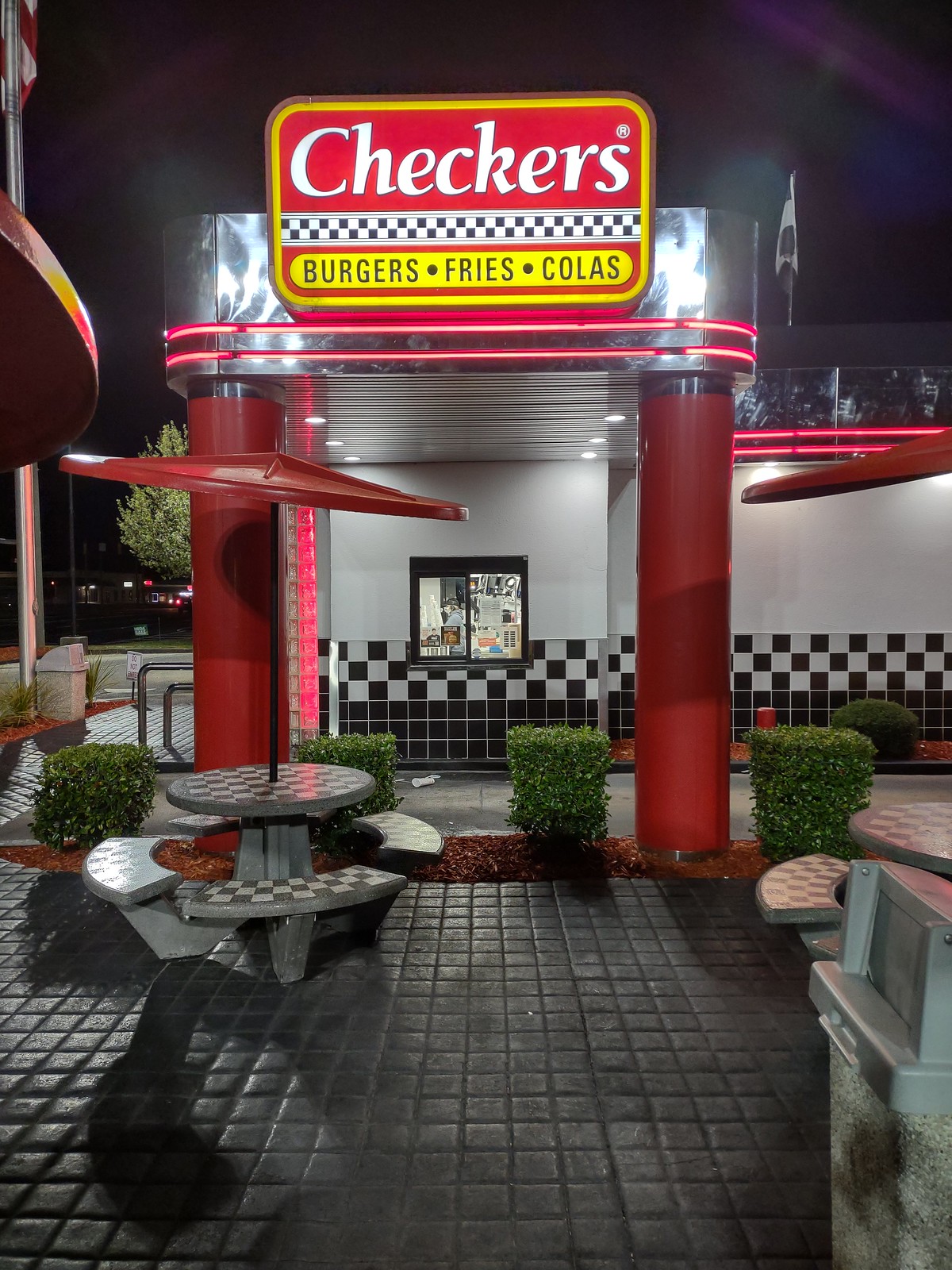This photograph, taken at night, captures the exterior of a Checkers fast-food restaurant. Dominating the top of the image is a large sign featuring bold white "Checkers" lettering on a red background, supported by two prominent red pillars. Below the main signage, there's a black and white checkered strip, and under it is a yellow oval stating "burgers, fries, colas." The building itself is a blend of white with black and white checkered trim around its base. The silver roof and the red columns supporting an overhang add to the restaurant's distinctive look. In the foreground, there's a clearly visible patio area furnished with circular tables and matching benches, all shaded by red umbrellas. A trash bin is located in the bottom right-hand corner, while green hedges frame part of the scene. In the background, distant trees and buildings add depth to the setting, and there's a noticeable drive-thru window area adjacent to the patio. The absence of people and vehicles adds a serene, almost still-life quality to the photograph.